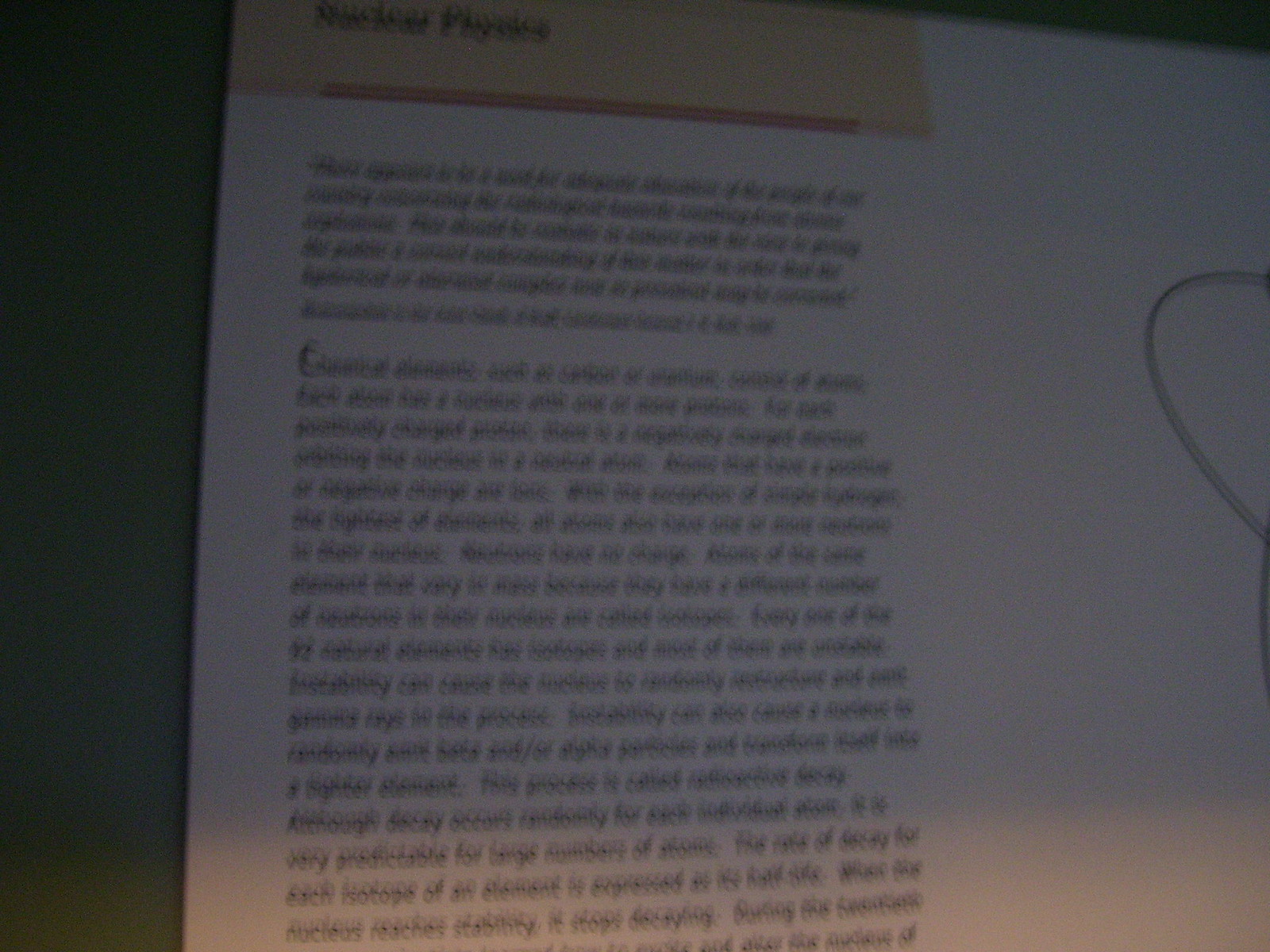This is a close-up photograph of a physics textbook page, taken in landscape format. The image prominently shows the top left section of the page with the heading "Nuclear Physics" in a yellow-highlighted area. Unfortunately, the photo is quite blurry and dark, making it difficult to read most of the text. Beneath the heading, there's a paragraph of text, written presumably about elements, but none of the words are legible due to the poor photo quality. To the right, a partially visible diagram with what appears to be an atom symbol can be faintly seen. The page lies on what appears to be a green surface, though the exact nature of the background is unclear. The overall impression suggests that the photograph was taken quickly and in low lighting, resulting in a very unclear and low-quality image.